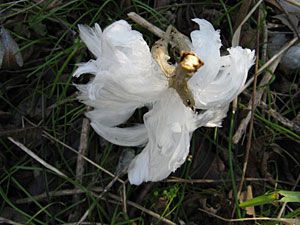The image depicts a wilted white flower with wispy, scraggly petals that almost resemble feathers. The flower appears to be a solitary bud, lying on a forest floor amidst twigs and grass. It looks like it has been separated from its original plant or tree, possibly clipped off, and now rests upside down, with its clipping point visible in the top right quadrant of the image. One can also notice a prominent blade of grass in the bottom right corner, adding to the scene's natural, woodland setting. The delicate, airy petals contrast sharply against the rough texture of the twigs and the soft greenery in the background.